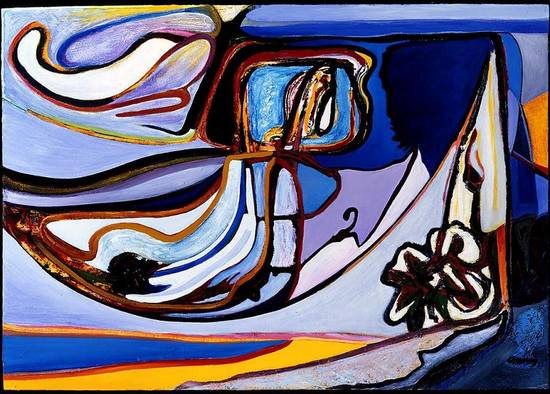This abstract painting, reminiscent of Salvador Dali's whimsical style and cubism, features a collection of vibrant and diverse elements immersed in a beach-like setting. Dominated by shades of blue, complemented by striking hues of purple, white, red, yellow, and gray, the image exudes a rich and colorful palette. At the bottom, the scene resembles a beach, with yellow sand and blue ocean waves gently meeting the shore. The composition includes an array of shapes—squares, circles, and more—scattered throughout, adding to the painting's complexity. A large, eye-catching flower stands prominently in the scene, alongside a figure who appears to be sitting next to a car or some other object, positioned on the right. Above and to the right, a formation that hints at a face, and below it, a shape that evokes the appearance of a coat hanger, add to the painting's intricate narrative. The entire composition, filled with whimsical lines and heavy, defining strokes, transports viewers to an imaginative and surreal seaside landscape.